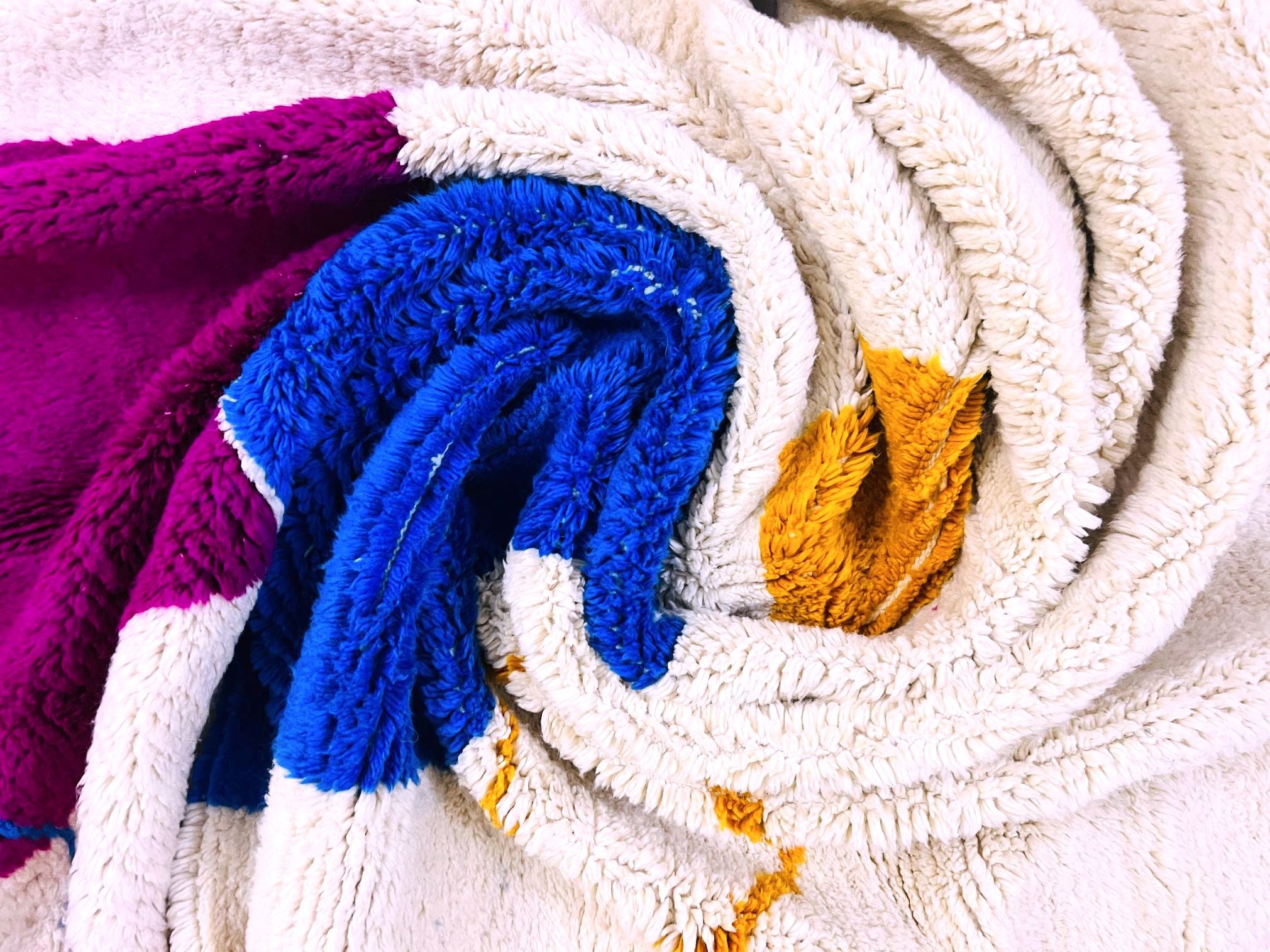The image captures a close-up of a luxurious, soft, and fluffy fabric that appears to be a blanket, though it could also be a beach towel or throw rug. This fabric has been intricately twisted and swirled into a spiraling pattern, creating a textured and cozy visual. Its primary color is a creamy off-white, with interspersed accents of deep blue, rich burgundy, mustard yellow, and a pinkish-purple hue, giving it a sophisticated and warm appearance. The material looks exceptionally soft and plush, likely made from microfiber or a similar fabric, with tufts and fine strands adding to its inviting, cozy aesthetic. The entire image is filled with this swirled fabric, and the intricate mingling of colors—creamy white, dark blue, burgundy, yellow, and pinkish-purple—offers a sense of warmth and softness.